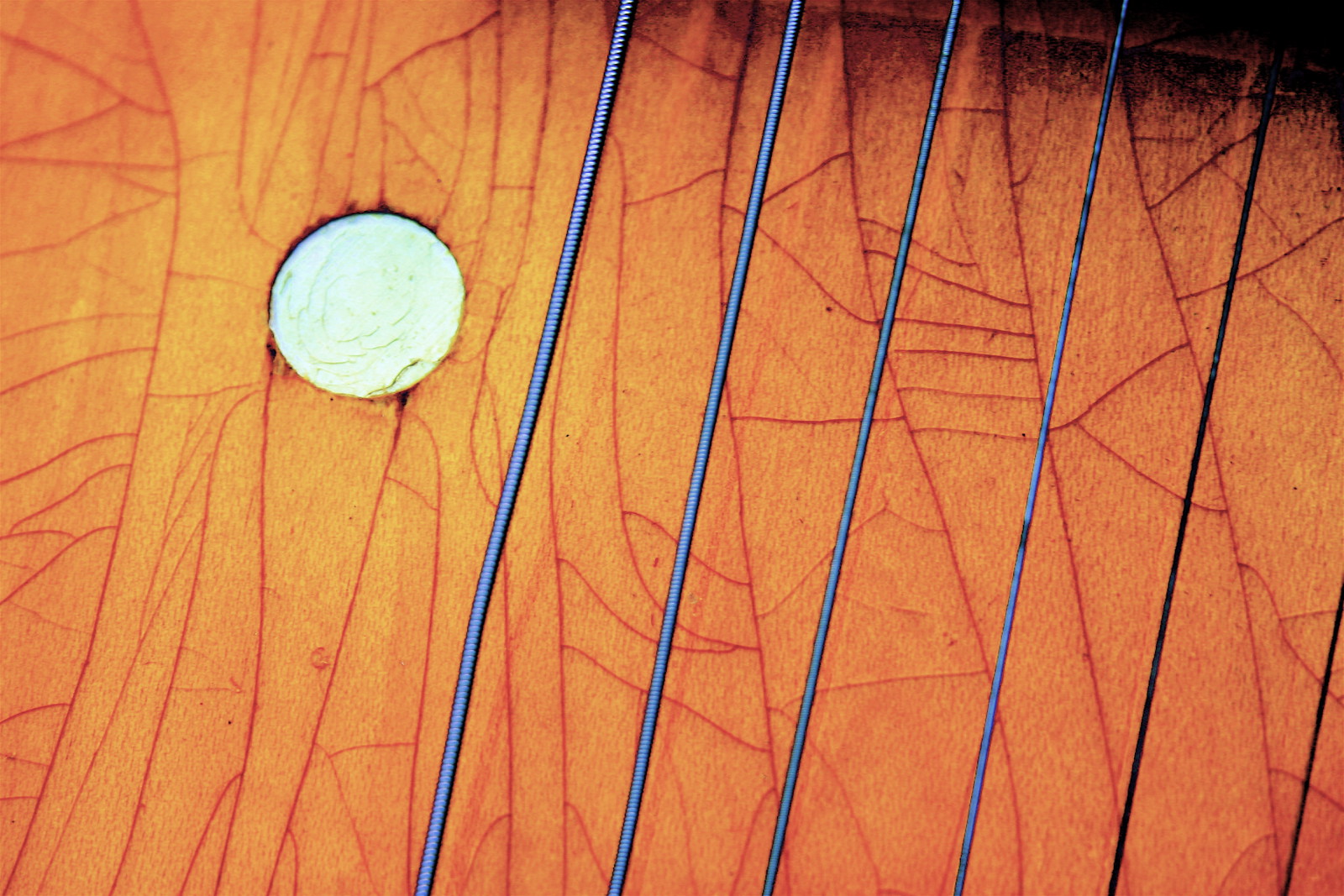The image appears to be a highly detailed close-up of a textured object, possibly wood or an acoustic guitar, with a complex pattern of colors and lines. The predominant color is a rich orange, with veins or wood grain patterns running through it in darker shades of brown. A significant feature in the top left corner is a yellow or white circular element that resembles a moon or a light source, casting a gradient that lightens the left side of the photograph. The light fades as it moves to the top right, where the color becomes a darker tan or brown with possible black scorch marks or stains. Additionally, there are several vertical bars or strings of varying colors—gray, blue, and black—angled slightly and contributing to the intricate design. This composition creates a visually dynamic image that blends organic textures with linear elements, illuminated by warm, vibrant hues.